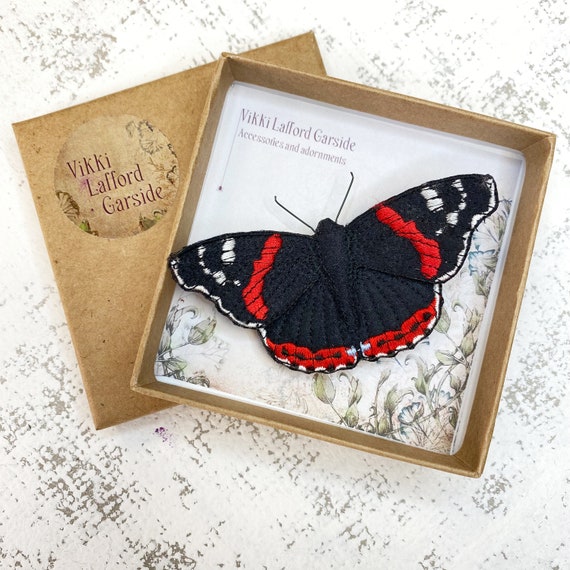This square-format color photograph captures a meticulously detailed accessory crafted by Vicky Lafford Garside. The central focus is a fabric butterfly pin, situated in an open, small jewelry box. The butterfly, which appears either crocheted or knitted, features black wings highlighted with vibrant orange, red, and white patterns akin to those of a monarch butterfly. The box enclosing this delicate creation has a brown cardboard hue and includes floral patterns, particularly visible in the bottom right of the case. The open lid, along with the exterior, prominently displays the name "Vicky Lafford Garside." The lid also provides the additional context of "accessories and adornments," confirming the nature of the product. The entire setup rests on a white table with subtle gray speckles, further enhancing the presentation of the butterfly pin.